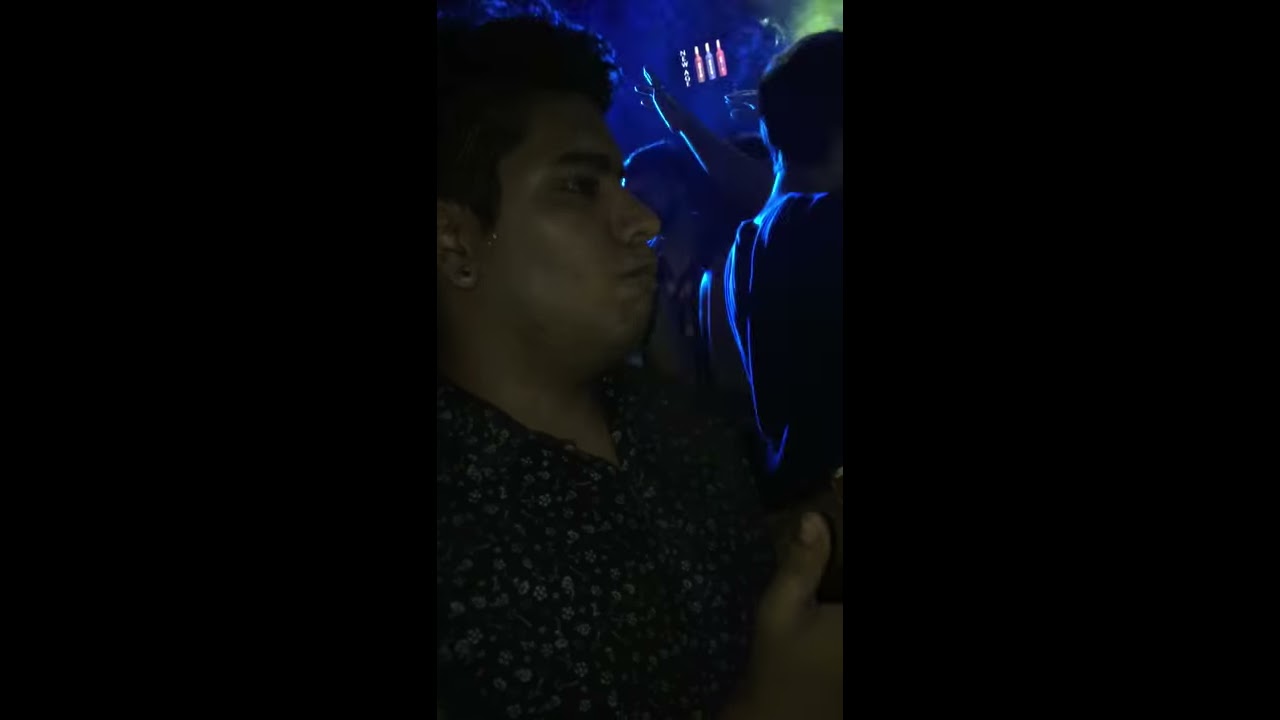The image depicts a man with short, curly, dark hair and an olive skin tone, in a side profile view. He is wearing a button-up shirt with intricate patterns, possibly resembling flowers, in black and beige-brown hues. The man is giving a thumbs up with both hands close together at chest level, his face appearing slightly scrunched and his lips closed. His earring is visible on the side. The scene around him is dimly lit, with noticeable blue and green lighting, creating a smoky, hazy atmosphere that suggests a nightclub or concert setting. Behind him, indistinct figures seem to be dancing, with one person notably raising an arm. In the background, a sign with the words "new age" and an illustration of three bottles is faintly visible, adding to the ambiance of the location. The left and right thirds of the image are shrouded in darkness, drawing focus to the central figure and the vibrant, busy environment around him.